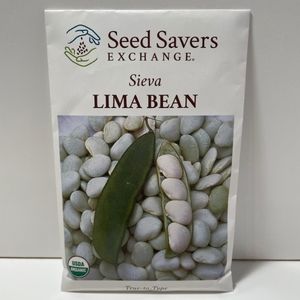This is a very small square black and white image depicting a bag of seeds for lima beans against a light background, possibly a table, and a gray wall behind it. The bag appears white at the top and features the text "Seed Savers Exchange" in black, with a logo to the left showing a blue hand pouring seeds into a green hand. Below that, it says "Sieva" and then "Lima Bean" in larger brown letters. The bottom part of the bag contains a photograph of a large pile of lima beans, with some displayed loose and others still inside the pod. There is also a dark object, possibly a leaf, to the left of the photograph.